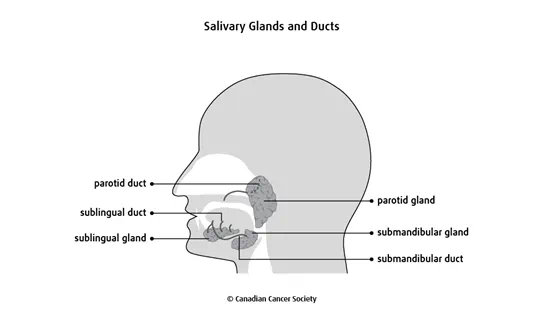The image is a detailed anatomical diagram, likely from a science textbook, labeled "Salivary Glands and Ducts" in bold black text at the top. It features a side profile illustration of a human head, oriented to the left, with a light gray color encompassing the head and neck, and white delineating the nasal cavities, mouth, and esophagus. The diagram meticulously labels and illustrates three key salivary glands and their corresponding ducts: 

1. The **Parotid Gland** and **Parotid Duct** are marked at the upper region, depicted as a spongy, rectangular mass with arrows pointing towards the area behind the throat.
2. The **Sublingual Gland** and **Sublingual Duct** appear in the lower part of the mouth, with arrows indicating their locations around the tongue.
3. The **Submandibular Gland** and **Submandibular Duct** are shown towards the bottom, with labels identifying their positions under the tongue and beneath the lower jaw.

Each gland and duct is carefully annotated, highlighting their positions relative to the head's anatomy. At the bottom of the illustration, "Canadian Cancer Society" is written in small black letters, indicating the source of the diagram.